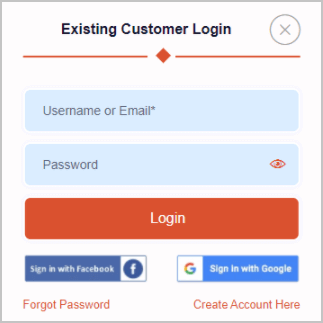The image features a square box outlined in faint gray. At the top center of the box, the text "Existing Customer Login" is displayed in bold black font. To the right of this text, there is a small white circle outlined in faint gray, containing an "X" in the center that is also faint gray in color. The middle section of the box showcases a red diamond shape flanked by two red vertical lines on either side. Below this, there is some space followed by a faint blue rectangular background. Within this rectangle, in gray text, is the phrase "Username or Email" accompanied by an asterisk (*). Beneath this input field, another faint blue rectangle contains the word "Password" in gray. The bottom section of the box features a bold red rectangle with the word "Login" in white text centered within it.